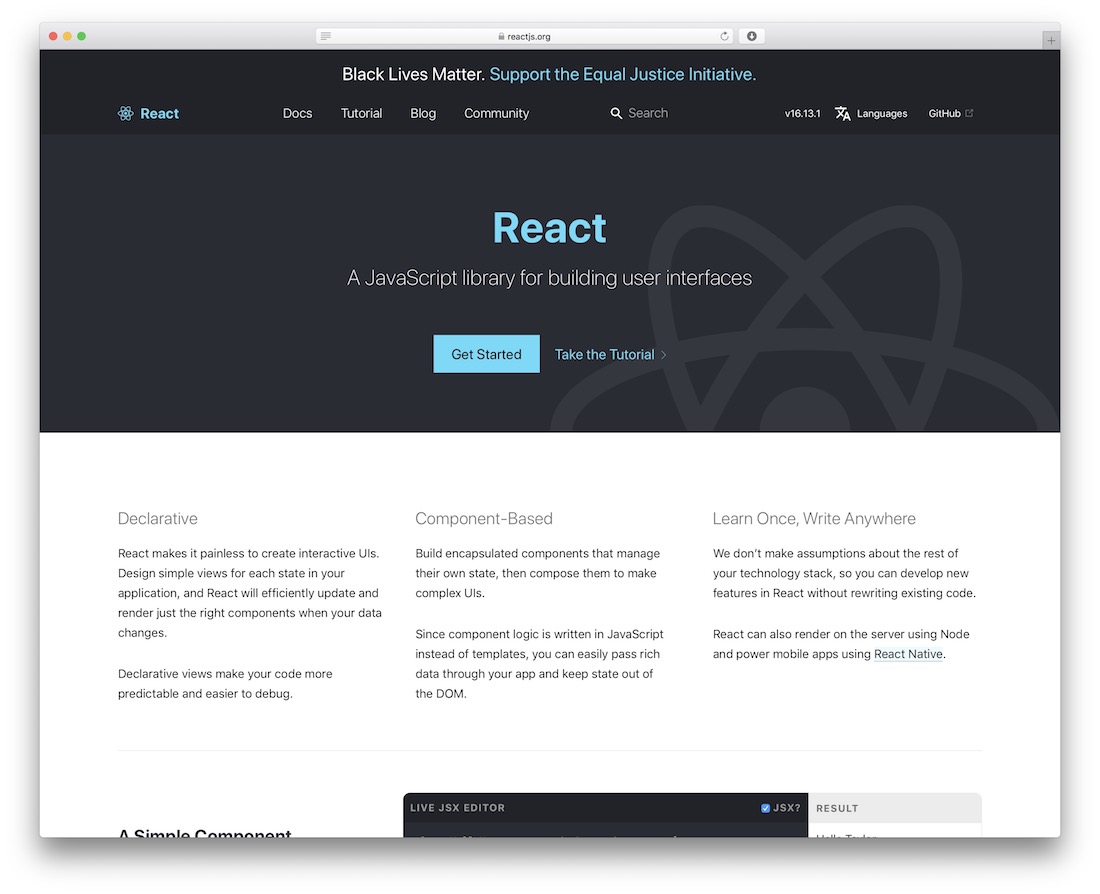This is a detailed screen capture of the homepage of the React website, accessible at reactjs.org. The image appears to show a browser window characteristic of Safari or a macOS browser. At the very top, there's a prominent header featuring the React logo situated in the top-left corner. Adjacent to the logo are navigation links labeled "Docs," "Tutorial," "Blog," and "Community," followed by a search bar with the placeholder text "Search." The version of React displayed is v16.13.1. 

To the far right, there are additional links for language options and the project's GitHub repository. Above this main navigation area, a banner stands out with a "Black Lives Matter" message, encouraging support for the Equal Justice Initiative, with the latter part of the text highlighted in light blue.

The main content features a prominent header image with the text "React – A JavaScript library for building user interfaces." Below this, there's a blue button with dark gray text labeled "Get Started" and a link that says "Take the Tutorial."

Further down, the page is divided into three columns highlighting key features of React: "Declarative," "Component-Based," and "Learn Once, Write Anywhere," each accompanied by brief descriptions. A thin line serves as a separator before the next section begins, where "A Simple Component" is visible as a heading, although much of this section appears to be cut off.